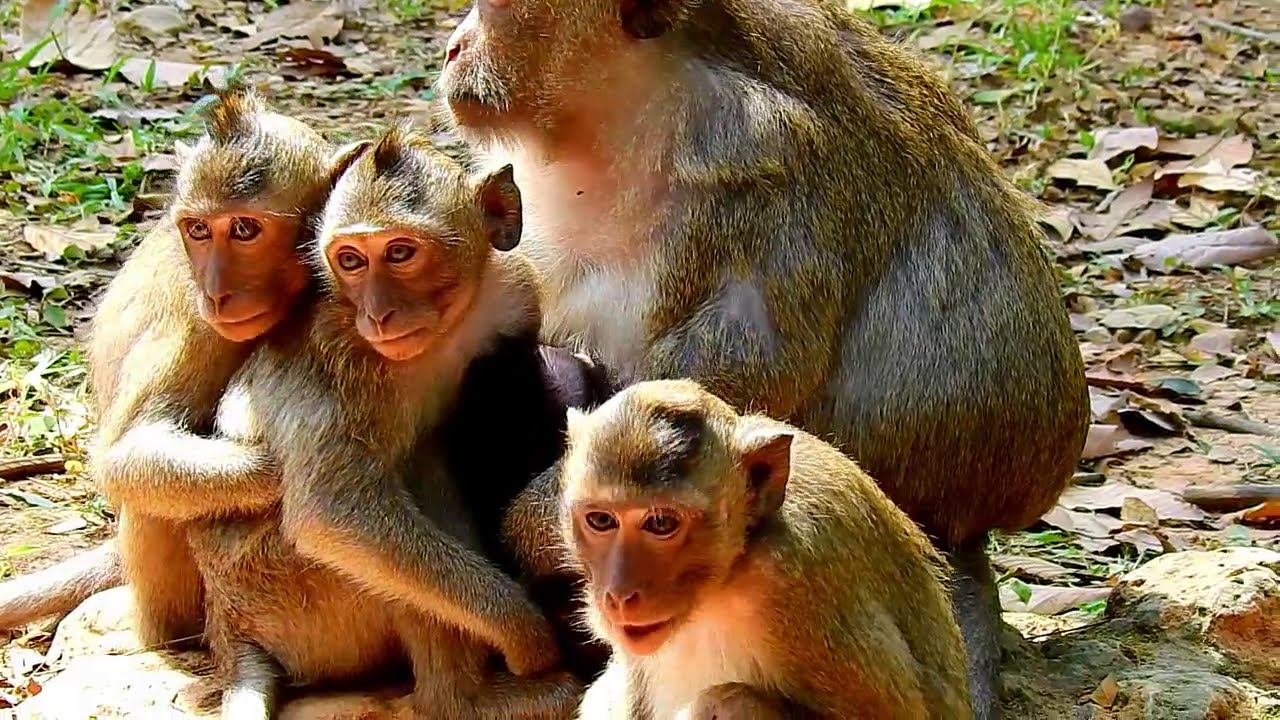This photograph captures a family of four monkeys in an outdoor natural setting bathed in sunlight. The ground, covered with dry leaves, green grass, small plants, and some rocks, creates an earthy, textured scene. Three smaller tan monkeys, with light-colored faces and white undertones on their fur, sit closely together in the foreground. One of the baby monkeys is hugging another, both looking towards the left, while the third monkey sits to their right, gazing downward and slightly to the center. In the background, a larger adult monkey, presumably their mother, is partially visible but her face is turned away, with the photograph cutting off just above her eyes. The sun illuminates their brownish-yellow fur, creating a warm, serene atmosphere in this natural snapshot.